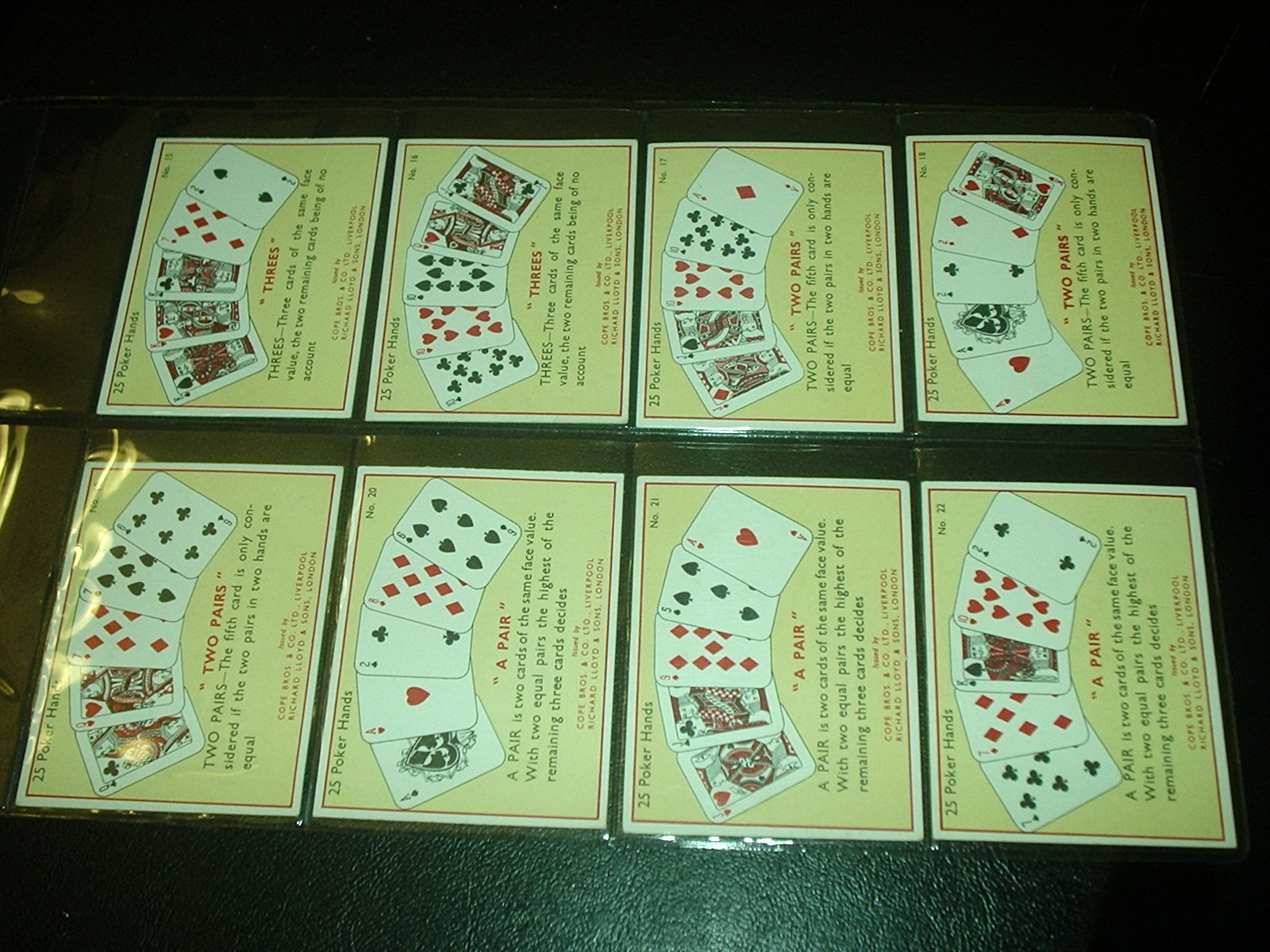The photograph showcases eight yellowish cards arranged in two rows, with four cards in each row. Each yellow card displays different combinations of poker playing cards and is intended to illustrate various poker hands. For instance, the bottom left card features a queen of clubs, queen of hearts, six of diamonds, six of spades, and six of clubs, illustrating what constitutes two pairs. To the right of this card, another card shows a different hand, identifying a pair. 

Beneath each displayed hand, there is red text indicating the type of poker hand shown, such as "two pairs" or "a pair." Additionally, black text provides a detailed explanation of what the hand represents. The overall purpose of the photograph seems to be educational, helping viewers understand the specific combinations and their meanings in the game of poker.